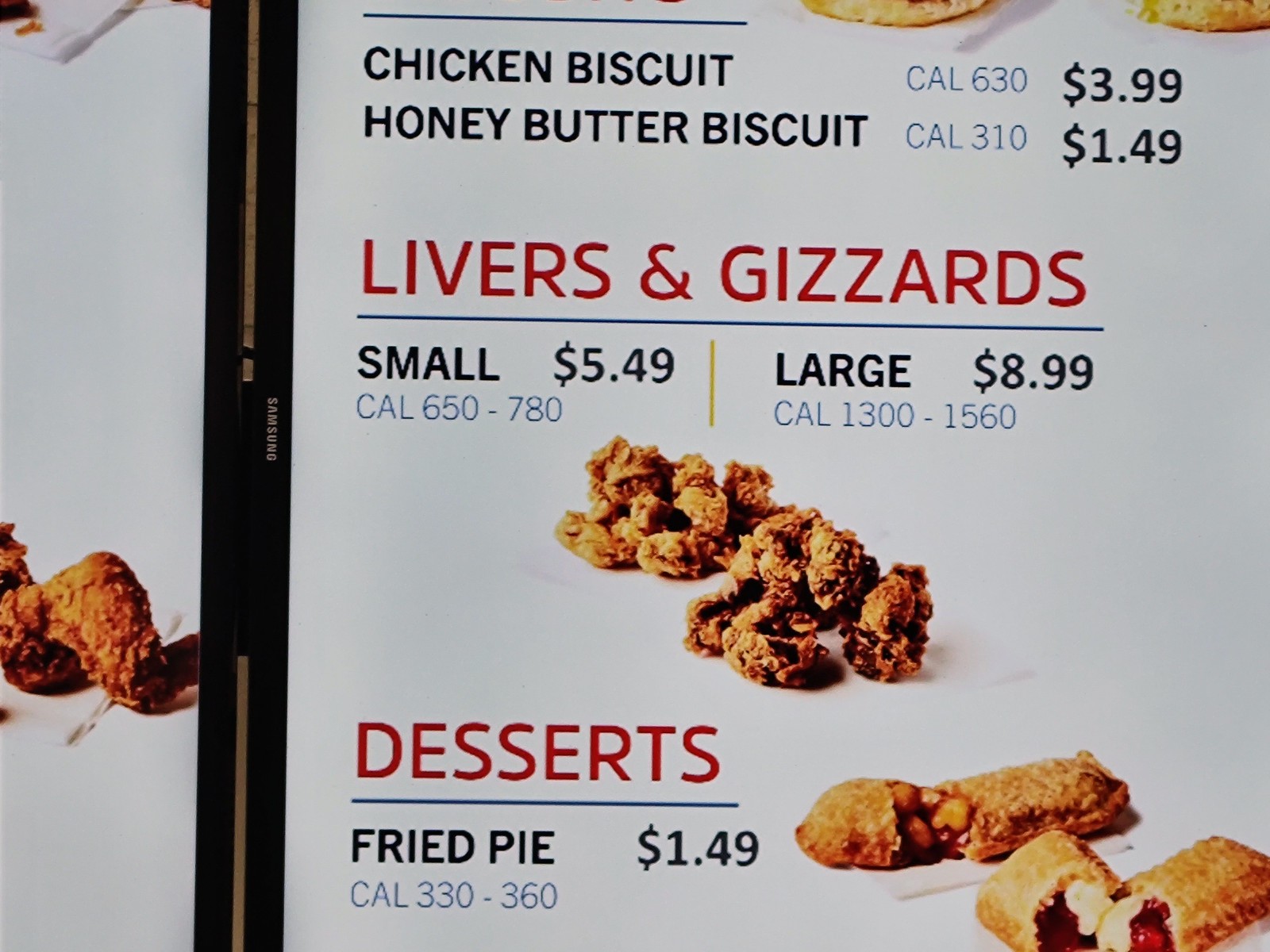This photo captures a segment of a fast-food menu, prominently displayed with various items and their respective caloric information and prices. At the top, the menu starts with:

- **Chicken Biscuit:** 630 calories, priced at $3.99.
- **Honey Butter Biscuit:** 310 calories, priced at $1.49.

Following this, there is a section titled "Livers and Gizzards":

- **Small:** Priced at $5.49, with a calorie range of 650 to 780.
- **Large:** Priced at $8.99, with a calorie range of 1300 to 1560.

A picture beneath this section visually represents the livers and gizzards for better appeal.

The dessert section lists:

- **Fried Pie:** Priced at $1.49, with calories ranging from 330 to 360. There are also images of two pie variations: one appears to be apple-filled, while the other seems to contain cherries and cream, although the latter is not entirely clear.

On the left-hand side of the menu, there are partial images of other menu items, but the text is cut off, rendering it unreadable.